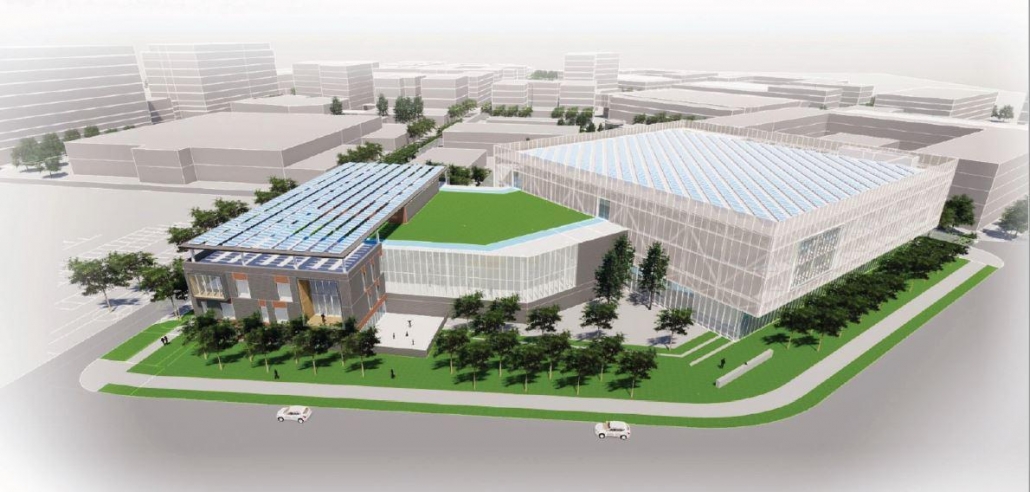This horizontal rectangular image is an architect's rendering of a proposed building complex, set in a landscaped green campus. Dominating the right side of the image is a large white building, accompanied by a lower, unusually-shaped white building in the middle, which features a courtyard in front of it. In front of these, a sidewalk meanders through an area adorned with numerous trees, meticulously placed on grassy patches interspersed with bushes. To the left, a gray building with distinct windows and roofing stands out, running along the side.

Beyond these key structures, the image suggests an industrial area, indicated by multiple two to three-story white buildings in the background. The upper left corner showcases much taller buildings, all adhering to a cohesive design theme with abundant windows. Notably, the middle building has a green rooftop, potentially an ecological feature. The combination of lush greenery, well-planned pathways, and modern architecture conveys an envisioned office building complex, where functionality meets aesthetic appeal.